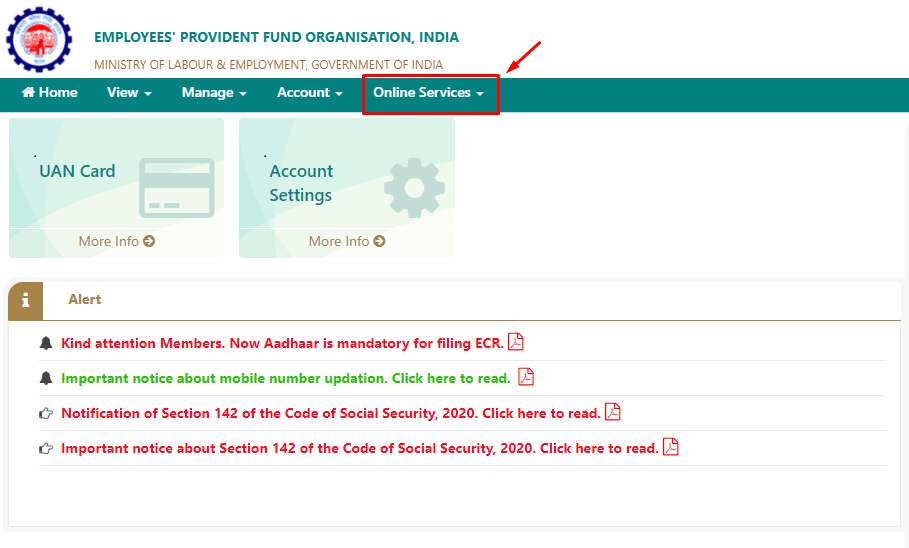This is a detailed screenshot of the online services page for the Ministry of Labor and Employment, Government of India, specifically showcasing the Employees' Provident Fund Organization (EPFO) interface. The screenshot is uncropped and features a predominantly white background accented with navy blue and sea blue labeled search bars and category bars. 

At the top left corner, the EPFO logo is prominently displayed, followed by a horizontal navigation bar offering various options, including "Home," "View," "Manage," "Account," and "Online Services." Notably, the last four options also function as drop-down menus, indicated by a downward-pointing white arrow.

Immediately beneath the navigation bar are two large, clearly marked buttons—one labeled "UAN Card" and the other "Account Settings." These buttons provide quick access to essential services. 

Below these buttons, there is a table titled "Alert" with multiple rows of critical updates:

- The first row, highlighted in red, reads: "Kind Attention Members: Now AADHAAR is mandatory for filing ECR."
- The second row, displayed in green, states: "Important Notice about mobile phone number updation, click here to read."
- The third row, in red text, announces: "Notification of Section 142 of the Code of Social Security 2020, click here to read."
- The fourth row, also in red text, says: "Important Notice about Section 142 of the Code of Social Security 2020, click here to read."

Each row provides crucial information and directives for employees, ensuring they stay informed about updates and requirements.

Overall, the design and layout of this page aim to facilitate user navigation and access to essential EPFO services and updates.